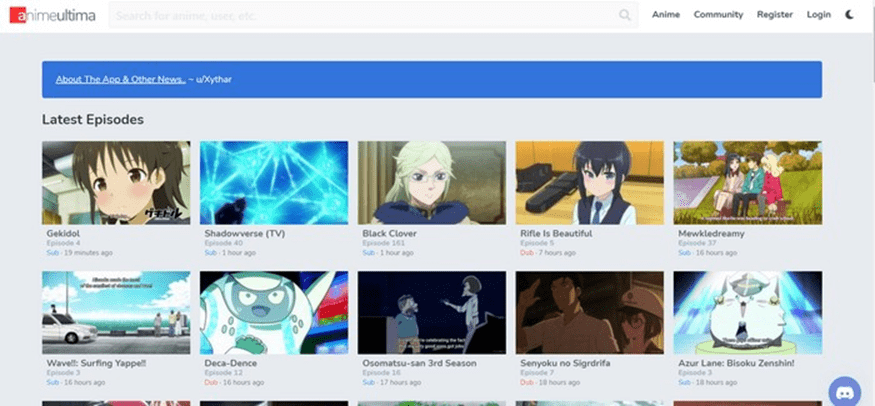The image is a color, landscape-format screenshot of the Anime Ultima website. The header prominently displays the site’s logo on the left, followed by a search bar that reads "Search for anime, user, etc." To the right of the search bar are navigational tabs labeled "Anime," "Community," "Register," and "Log In." Just below these tabs, options for "About the App" and "Other News" are available for more information.

The main content of the page showcases the latest uploaded episodes of various anime series. The titles and their respective episode details are visibly listed. Among these are:
- Gekidot, with Episode 4 recently added 19 minutes ago,
- Shadowverse with Episode 40,
- Black Clover with Episode 101,
- Rifle is Beautiful,
- Mukledreamy,
- Wave, Surfing,
- Yap,
- Decadence,
- Osomatsu-san,
- Senyoku no Sigurdrifa,
- and Azur Lane.

The interface is structured to provide users with quick access to recent updates and extensive anime content, emphasizing user engagement and ease of navigation.